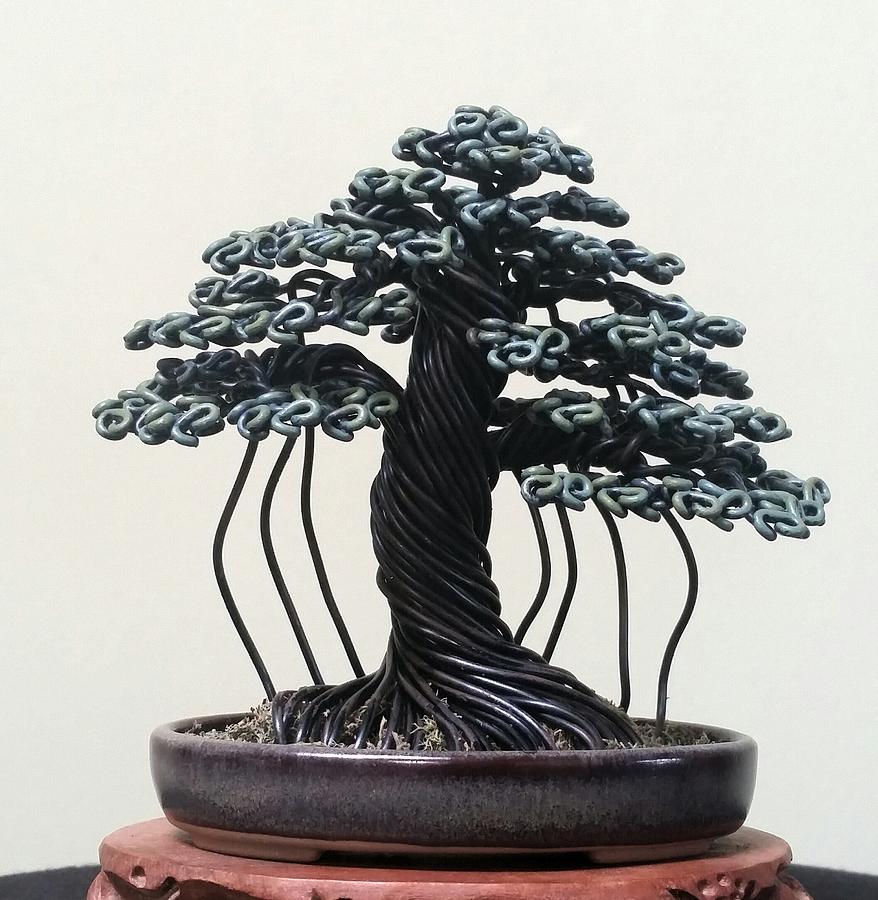The photograph features an intricately crafted bonsai tree statue that serves as a piece of art. The backdrop is a beige-colored wall that contrasts subtly with the brown, intricately carved wooden platform on which the statue is displayed. The bonsai tree is housed in a shallow, black-brown ceramic pot that resembles a wide dish. The tree itself is artistically fashioned from dark brown wires that are intertwined to form the trunk and branches, giving the sculpture a dynamic and textured appearance. The leaves of the tree, shaped like tiny "E" figures, are crafted from a shiny metal, possibly silver or teal, adding a contrasting pop of color and detail. The base of the tree features what looks like coconut coir or moss, enhancing its lifelike quality. Some untwisted wires extend from the branches to the base, appearing to support the structure. This art piece masterfully combines various materials to mimic the natural elegance and complexity of a real bonsai tree.